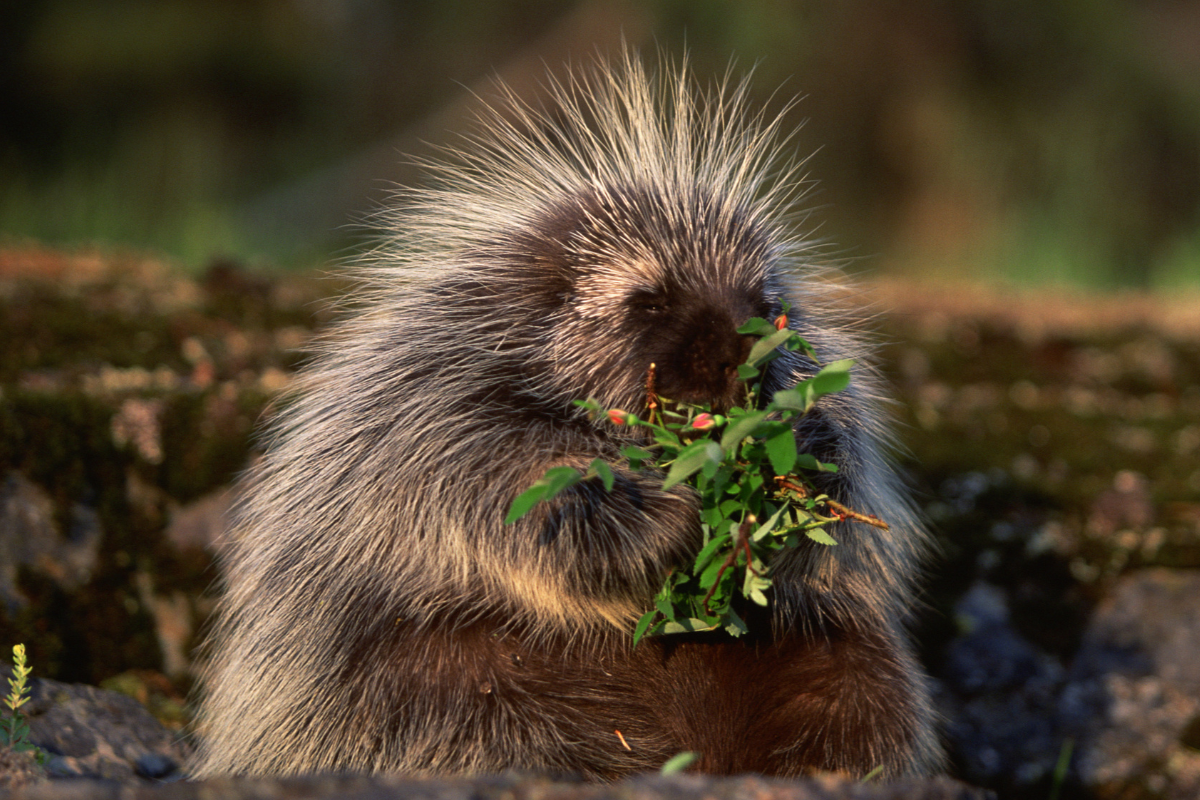This close-up, professional photograph features a well-defined hedgehog, characterized by its brown and white fur which sticks up in little points on top of its head. The hedgehog's small eyes peer out as it sits with a rotund belly, holding a piece of shrubbery in its paws. The greenery it holds is dark green with tiny leaves and little red flowers, suggesting it may be part of the hedgehog's meal. The bright, nice day adds to the vividness of the scene, though the background of dirt and plants is intentionally blurred, directing full attention to the content and texture of the hedgehog’s fur and its engaging pose.